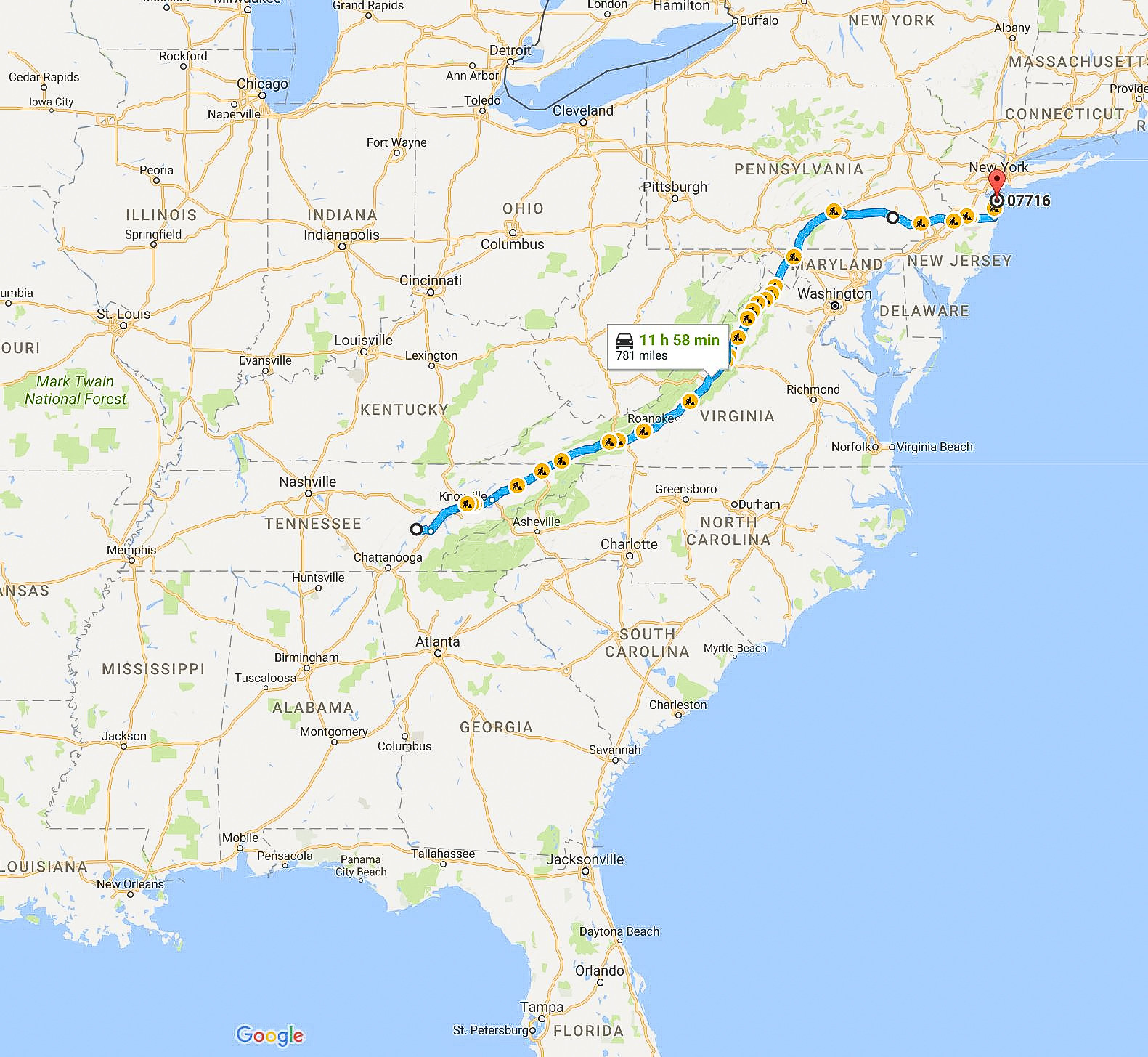This image depicts a detailed map covering the majority of the United States, specifically highlighting the area from Missouri, Iowa, and Arkansas in the west to the eastern coastline. The map features a prominent display of interstate highways marked in red, crisscrossing the nation. The source of the map is likely MapQuest or Google Maps, evident from the layout and style.

A highlighted route is visible, starting in Tennessee, just north of Chattanooga and slightly west of Knoxville. The destination appears to be somewhere in Pennsylvania or New York, near the Atlantic Ocean. The annotations on the map indicate a calculated driving time of 11 hours and 58 minutes to cover a distance of 781 miles.